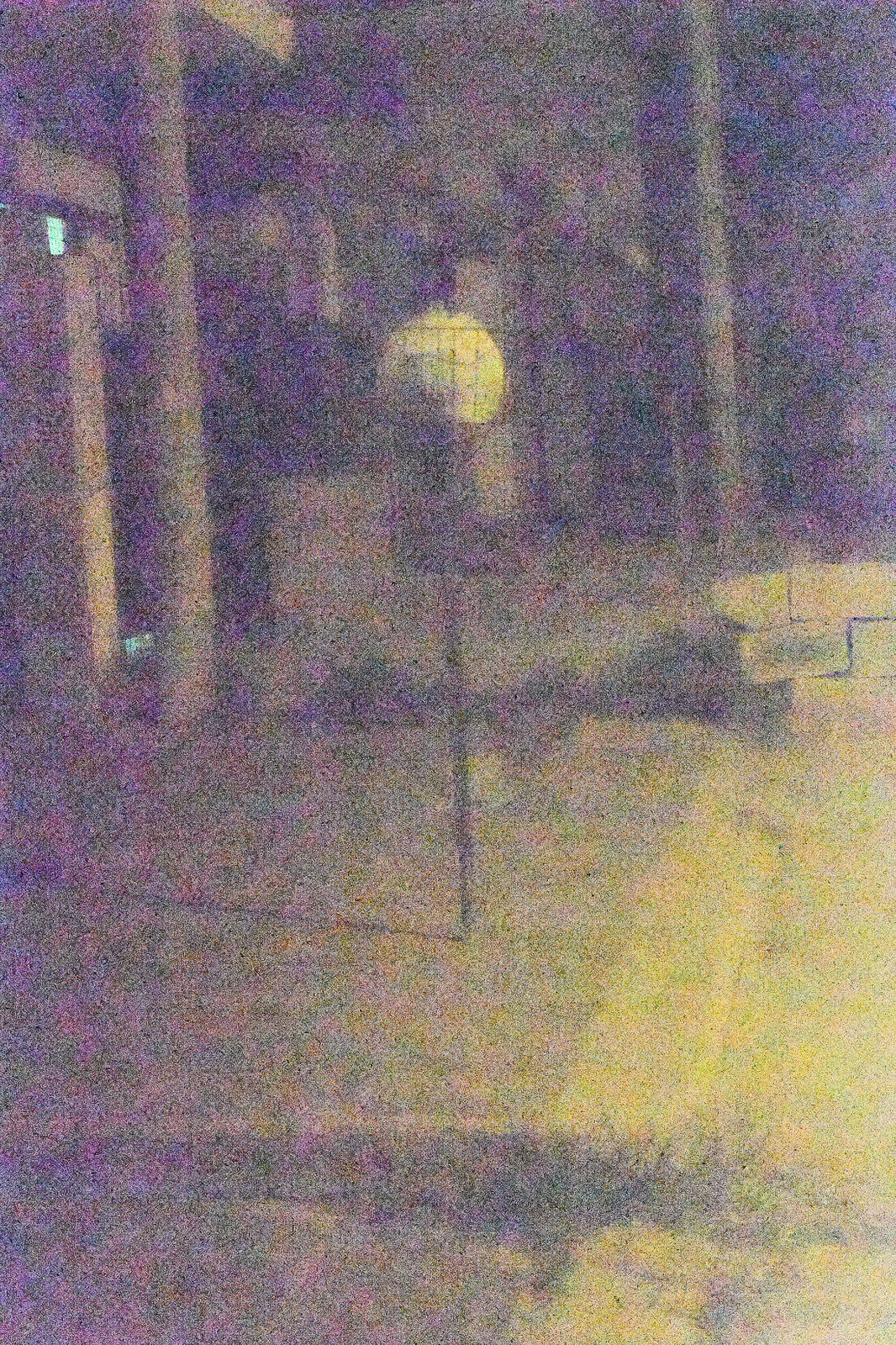This grainy, faded black and white photograph features a weathered sidewalk with thick tufts of grass sprouting between the cracks. A metal pole rises from the middle of the sidewalk, topped with a white, round object perched on a square, black base. To the left, a tall tree or pole stretches upwards, partially obscuring a structure that appears to be a house or building. This building has a small, square window near the roof, hinted at by its faint blue hue. In the background, the skeletal outlines of trees can be seen casting shadows. At the edge of the sidewalk, a yellow-painted curb separates the walkway from the road.